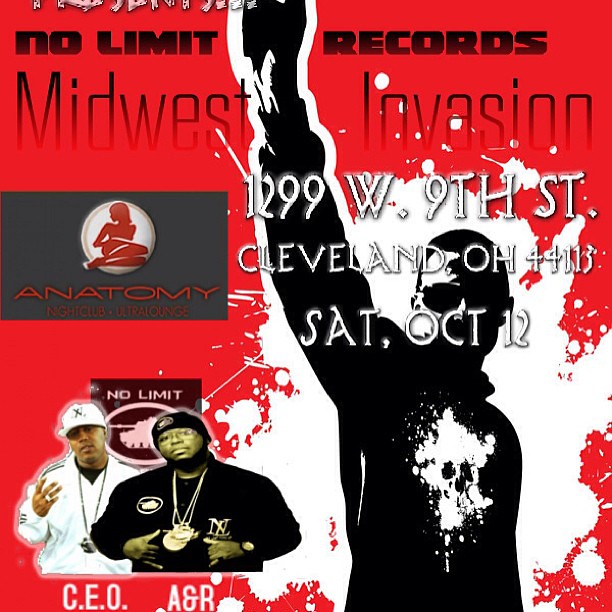This vibrant red advertising poster promotes "No Limit Records Midwest Invasion" event. Dominating the center-right, a graphic of a black man wearing sunglasses and dressed in black raises his fist against a white splash on his shirt, with white splashes surrounding him. Flanking him to the left are two men on the bottom left corner: one is a black man in a white t-shirt, white baseball cap, white jersey, and a large medal identified as the "C.E.O.," and the other, a black man in a black stocking cap, black sweatshirt, and two medals, identified as the "A.N.R." Above them is the "No Limit" logo, and further up, within a circle, is a woman in red with “Anatomy” written underneath. The top section of the poster displays the event details in black text: "No Limit Records Midwest Invasion," "1299 West 9th Street, Cleveland, Ohio 44113," and "Saturday, October 12th." The poster’s graphic elements and text collectively beckon viewers to this lively club event.